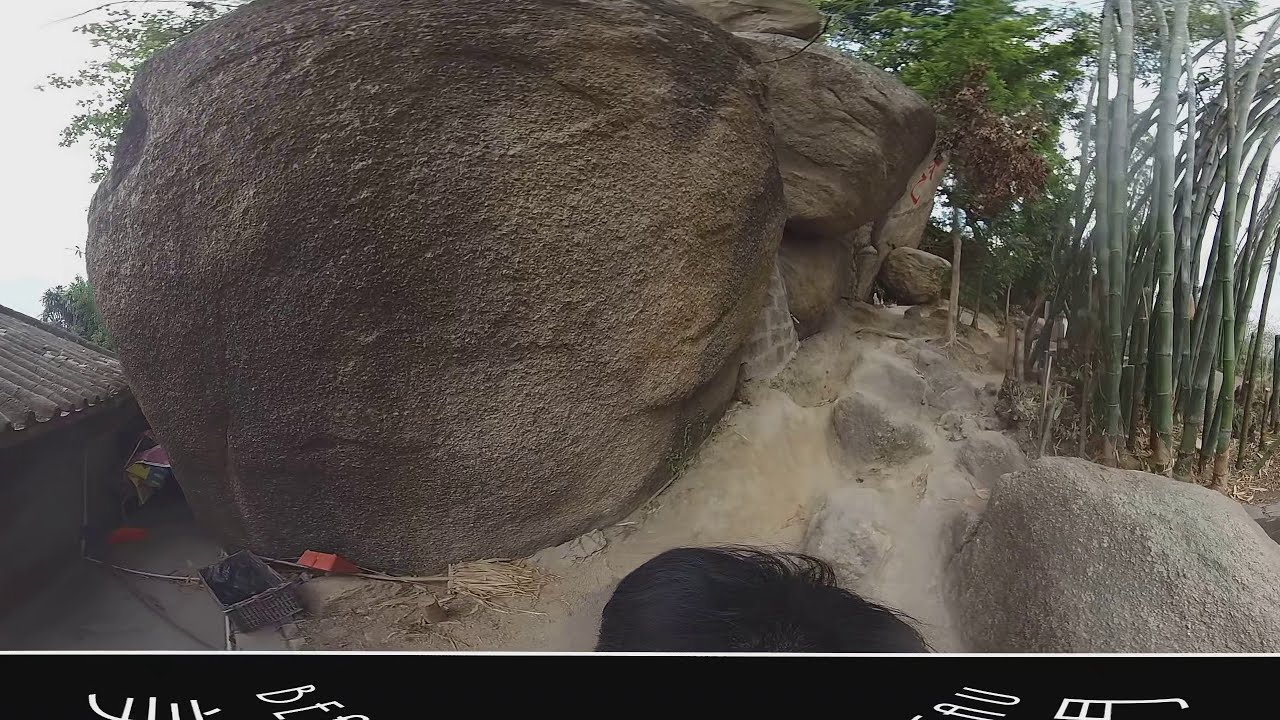The image captures an outdoor scene dominated by a series of large, smooth boulders. In the foreground, two connected boulders are prominently displayed; the closer one is smoother and rounder while the further one is more irregular and jagged, featuring holes and red graffiti. Nearby, a smaller boulder sits beneath the graffiti. At the bottom of the image, there is a black strip outlined in white with partially visible white letters spelling "B-E-A-U," though the writing is largely cut off.

In front of the largest boulder, there appears to be a handmade wooden crate, though it’s not very clear. The background includes a mixture of bamboo-like stalks and green trees, contributing to the lush ambiance of the scene. To the left, a gritty concrete wall connects with a rustic corrugated tin roof situated close to the boulders. Additionally, the bottom middle of the image reveals part of a person's head and hair.